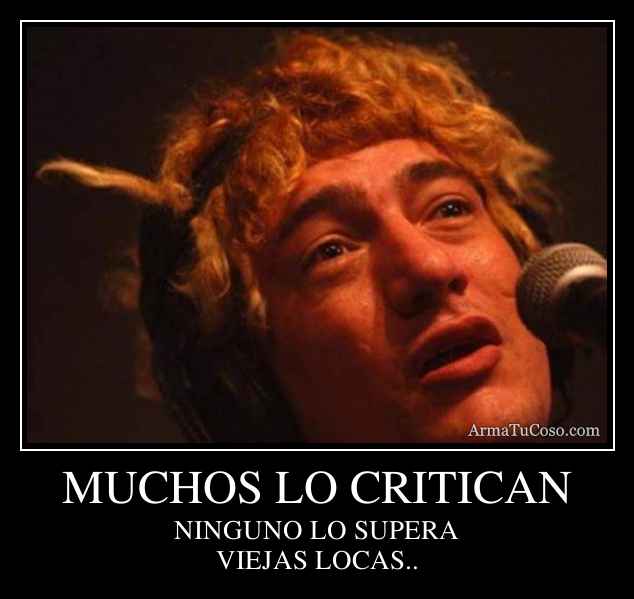The image depicts a graphic photograph of a male singer with curly, golden-blonde hair, singing into a silver microphone positioned to the right side of his face. The singer's face is shown in close-up within a white-bordered rectangle against a black background. Below the photograph, the website "armatucoso.com" is displayed in white text. Beneath this, more text follows, also in white: "muchos lo critican," and further down, "ninguno lo supera." The entire graphic stands out sharply due to its black background, and the detailed features emphasize the singer's expressive performance and the accompanying impactful text.